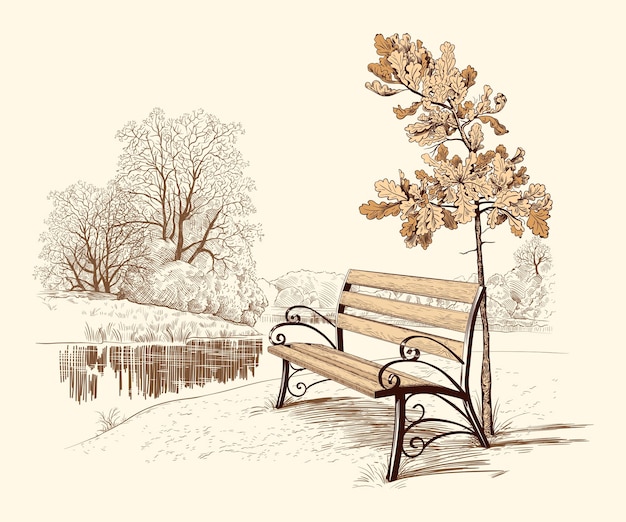This detailed drawing, reminiscent of an illustration from a book, depicts a serene park setting by a river or lake, bathed in soft pastels and light tans. The centerpiece is a wooden bench, characterized by three slats on the backrest and additional slats on the seat. The bench features ornate black iron armrests and curly Q braces on the feet. Positioned directly behind the bench is a small sapling with brown leaves, indicative of mid to late autumn. The grass, rendered in pencil, appears gray, blending seamlessly into the tranquil scene. Across the river, the opposing shore is lined with larger, somewhat barren trees with sparse leaves, their muted reflections abstractly captured in the water. The entire picture exudes a warm, pale yellowish tinge, creating a cohesive, calm ambiance.